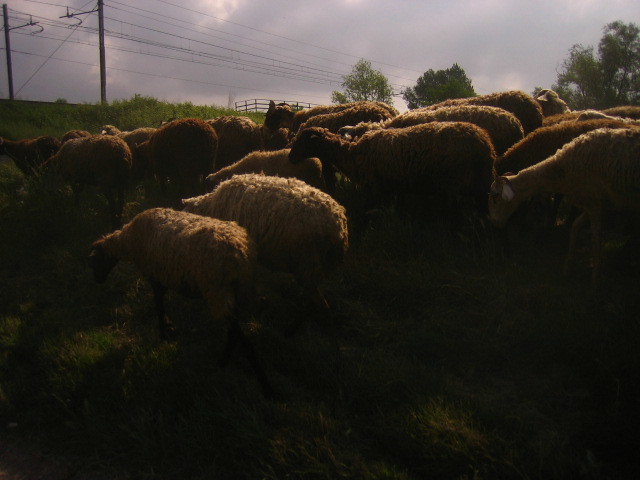The photograph captures a herd of around 20 to 30 sheep grazing in a field of very tall, uncut grass on an overcast day. The sky is filled with dark, rain-laden clouds, casting a muted light across the scene. The sheep exhibit a variety of colors, with some having dark chocolate brown wool, while others display hues ranging from cream to off-white. Notably, several of the sheep have distinctive black faces and legs extending from their matted wool bodies. The sun manages to peek through the clouds just enough to cast light on the tops of a few of the sheep, leaving their lower bodies in shadow and making it hard to discern their feet and the base of the grass blades.

In the background, we see the tops of several green trees and noticeable infrastructure, including telephone poles with wires stretching into the distance and low-slung metal gates, suggesting a nearby road or railway line. The sheep appear to be moving from the right side of the photograph, receding into the background toward the left, seemingly indifferent to any potential noise from nearby traffic or trains. This pastoral scene conveys a sense of tranquility despite the gloomy weather.